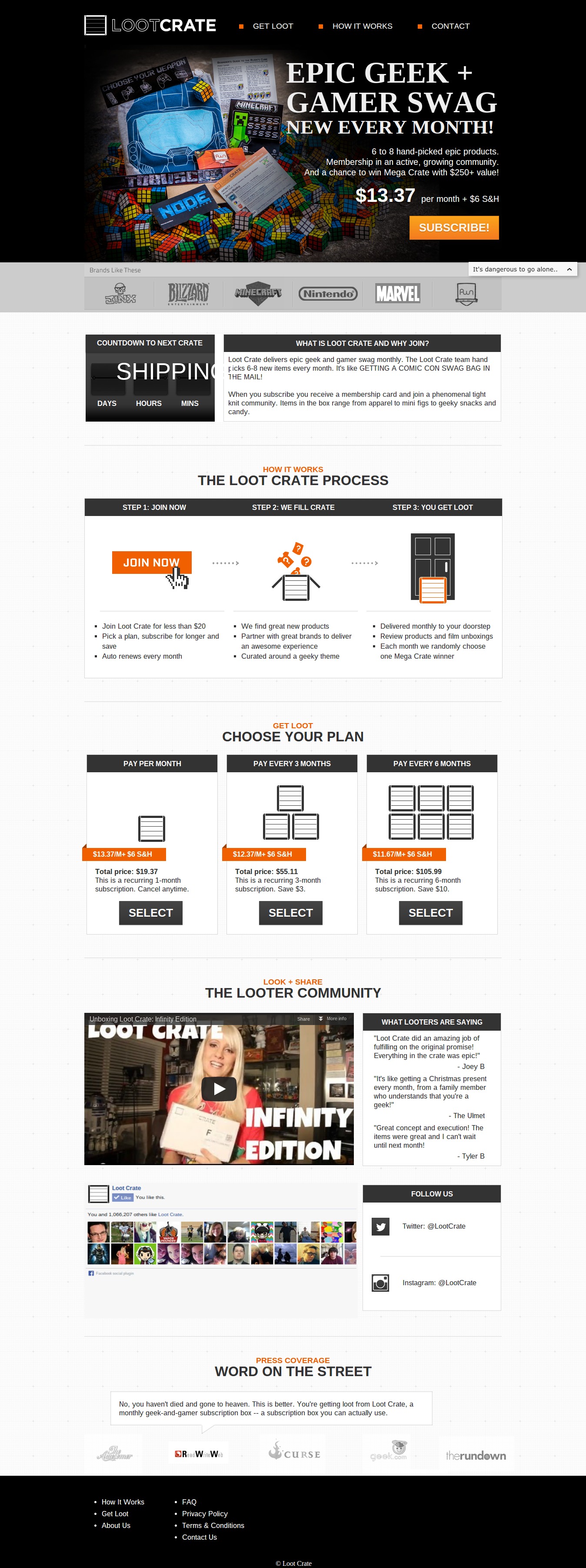Screenshot Description: 

The screenshot captures a web page, possibly belonging to an online gamer community or a site retailing products targeted towards gamers. The top portion features a black rectangular bar adorned with various brightly colored icons, though they are indistinct. This black bar likely serves a navigational or informational purpose. 

Prominently displayed in white text on this black background are the words "Epic Geek and Gamer Swag, new every month" with a price of $13.37 mentioned below. Although there is some very fine print in white on the black background, it's unreadable in the image.

Beneath this headline, there is a detailed explanation regarding the subscription service, which appears to be for a monthly loot crate delivering assorted items. This section includes diagrams presented in black and white, each highlighted with an orange bar, though the specifics of these diagrams are too small to decipher.

At the bottom of the screenshot, there is what seems to be a promotional video for the product accompanied by a chat box, suggesting an interactive feature or customer support option on the web page.